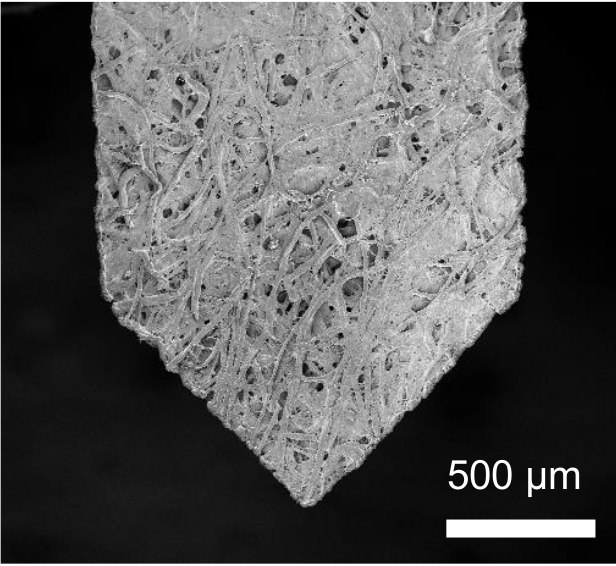The photograph depicts a highly magnified black and white microscopic image centered on a distinct, somewhat triangular shape that tapers to a point at the bottom, resembling the form of a men's necktie. The object appears gray due to the monochromatic presentation and is characterized by a network of intertwining fibers or threads, creating a detailed texture replete with black speckles and ridges. Situated in the bottom right corner of the image is a label in white text reading "500 micrometers" in a rectangular white box, indicating the scale of the magnification. The black background of the photograph accentuates the structural details and complexity of the specimen, giving it an almost abstract, yet intricately detailed appearance akin to a Jackson Pollock painting.